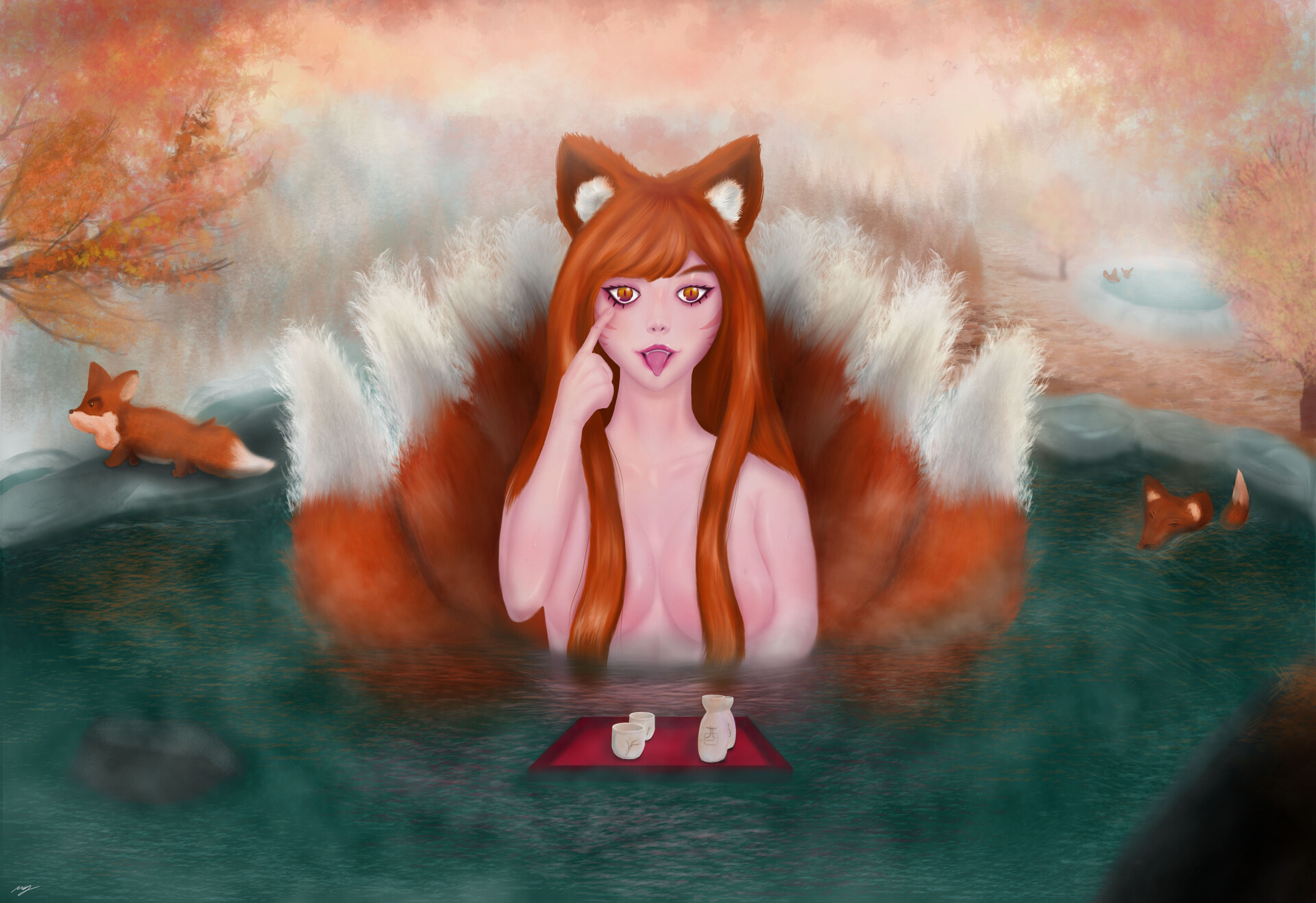The image is a detailed digital drawing of a woman with long, reddish-brown hair that falls over her chest, strategically covering her nipples. She has large, pointed ears that are brown with a white center, resembling fox ears, which blend seamlessly into her hair. The woman has an intriguing crimson eye, which she points to with her red-tinted hand while sticking out her tongue playfully. Behind her, multiple bushy, brown fox tails with white tips fan out, creating a striking, peacock-like effect.

The setting appears to be a small, bluish body of water, possibly indicating a lake or pond. On either side of the woman, there are brown foxes; one seems to be swimming on her right, while the other is positioned on the bank to her left. The background features trees with orange foliage, suggesting an autumn scene. Additionally, a floating red serving tray is present in front of her, with two sake cups and a small serving pitcher, adding an interesting, cultural element to the composition.